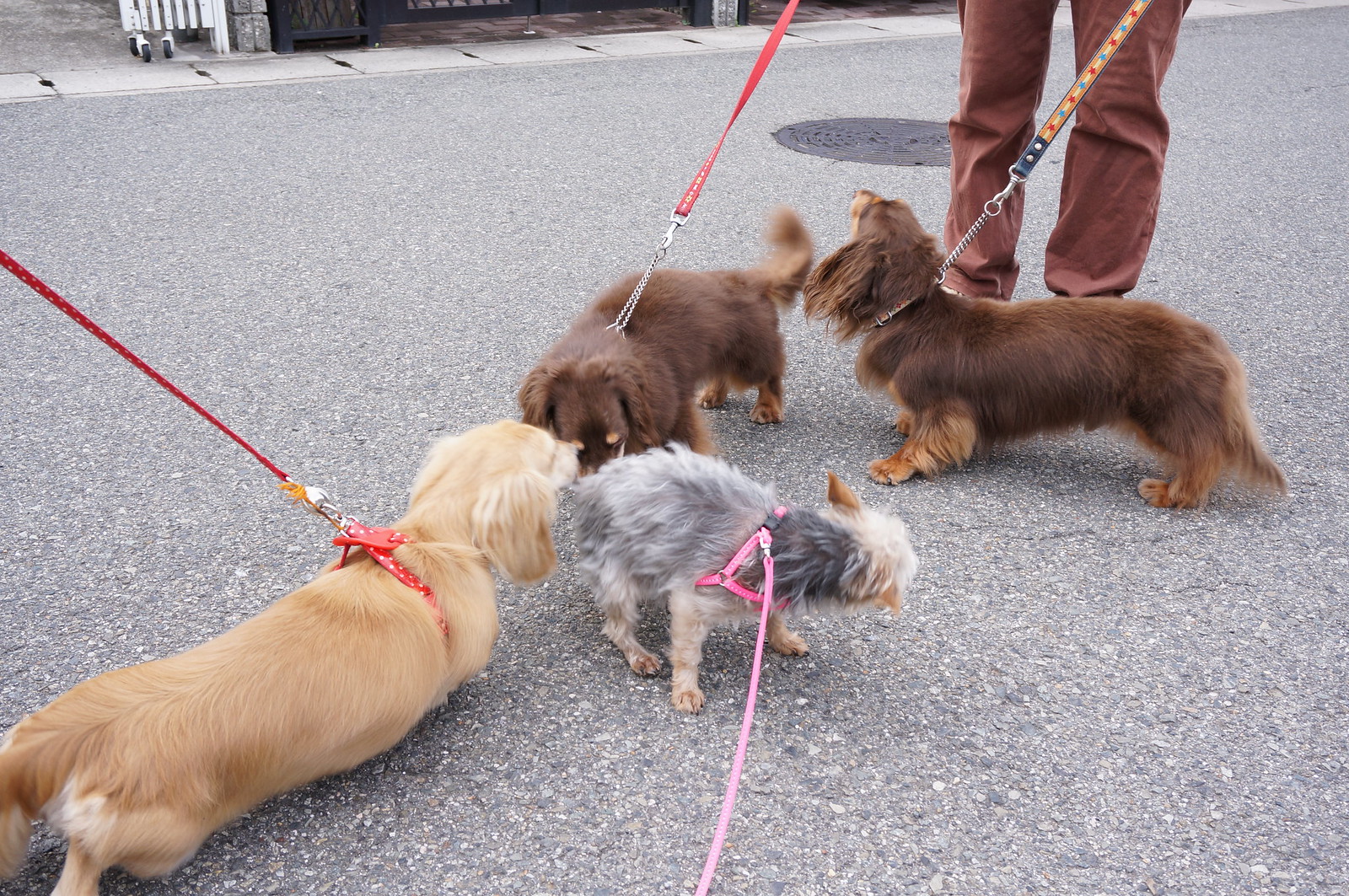This is a color photograph depicting a group of four small dogs on a grey pavement, possibly in an urban area. The pavement features a covered round manhole near the upper edge of the image, bordered by a line of bricks or slates and a notable black shadow. The dogs, all on leashes, seem to have momentarily paused to interact with each other. 

The dog on the bottom left is a light beige, almost sandy-colored, long-bodied dog on a red leash and harness, positioned with its back legs slightly raised. In the center, there's a small grey and cream terrier-like dog, sporting a pink collar and leash, its head turned away from the camera. Two similar-looking dark brown dogs, distinguished by lighter brown legs, feet, and slightly lighter faces, are also present. One brown dog has a red leash with a metal chain, and the other has a multicolored leash, held by an unseen individual wearing brown pants. The interaction and conditions suggest a casual encounter on a concrete street, devoid of visible shoppers or other distractions, making the dogs the focal point of the scene.